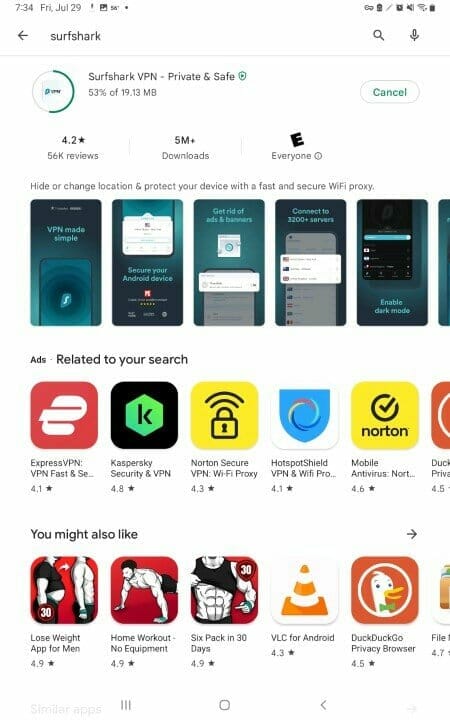Caption: On Friday, July 29th, at 7:34, the screen displays a variety of app icons and information. Featured prominently is a download status for Surfshark VPN, which advertises private and safe internet browsing with a fast and secure Wi-Fi proxy. The download is at 53%, with 19.13 megabytes remaining. Surfshark VPN is rated 4.2 stars from 46,000 reviews and has over 5 million downloads. It's suitable for everyone. Text also highlights the benefits of changing your location and protecting your device. Additionally, there are mentions of other apps and services including ExpressVPN, rated 4.1 stars, a 4.6-star rated mobile device, a 4.9-star rated home workout app promising a six-pack in 30 days, and DuckDuckGo for secure browsing on Android devices.